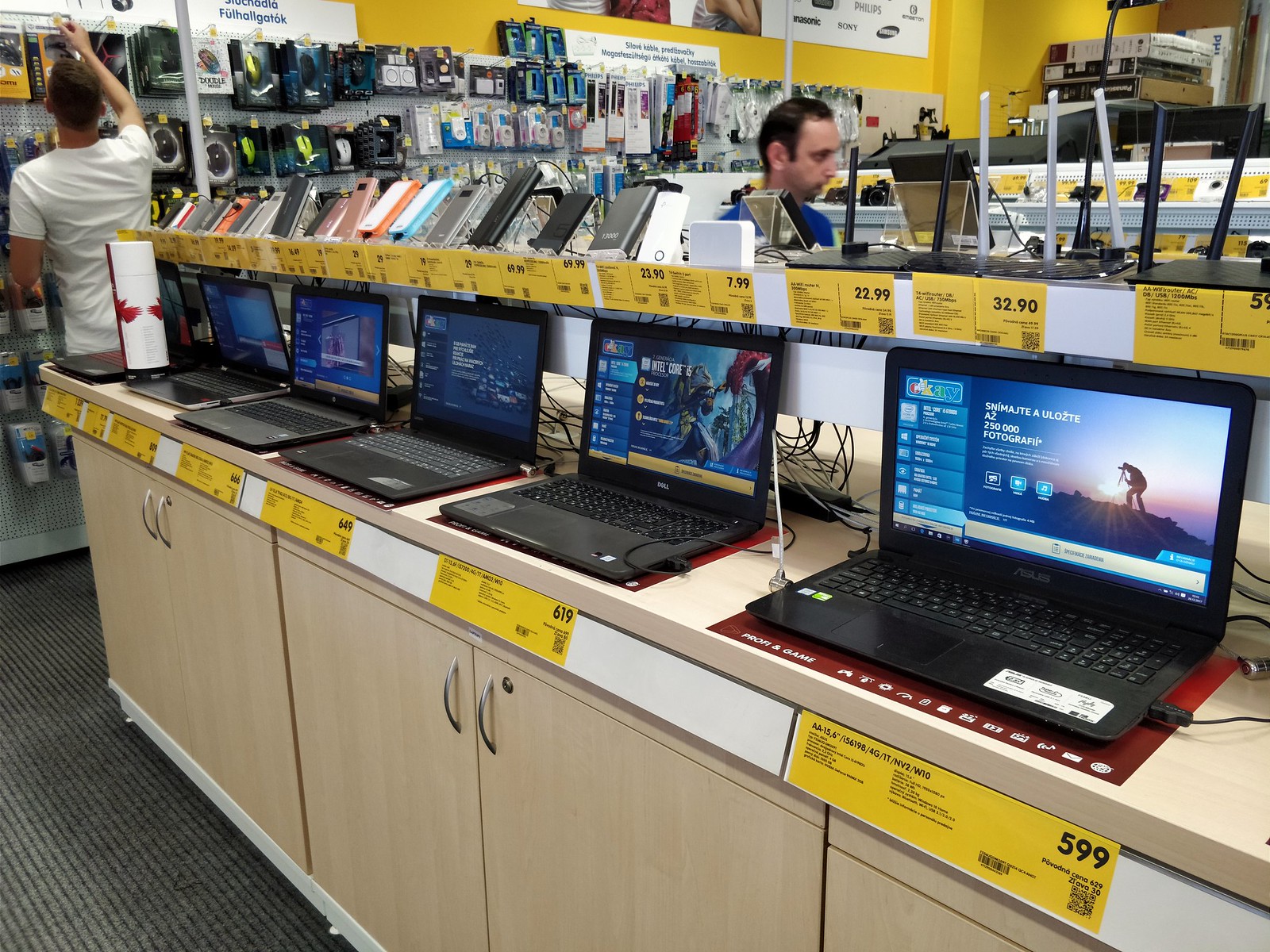The photograph captures the inside of what appears to be a Best Buy or a similar electronics retail store. At the forefront, there is a display of several different Microsoft laptops, neatly arranged side by side on a beige counter that mimics natural wood. These laptops feature yellow rectangular price tags in front of them, with prices like $599, $619, and $649 clearly visible. Notably, the clearest laptop's price tag displays "AA156" and is priced at $5.99 with detailed information in what seems to be a Scandinavian language.

Beneath the laptops, the counter has cabinets with silver arched handles and keyholes, suggesting secure storage. In the background, the store features racks of various electronic accessories, possibly including computer mice, power banks, or phone cases. 

Two men can be seen interacting within the store. One man, with short dark hair and a blue shirt that resembles a Best Buy uniform, is partially obscured by product shelves. Another man, wearing a white t-shirt and also with dark hair, is reaching up to grab something from a shelf that contains more accessories.

The environment reflects a bustling retail space typical of a Best Buy, characterized by a mix of colors including yellow, black, gray, and beige, with bright lighting enhancing the visibility of both products and informational tags.